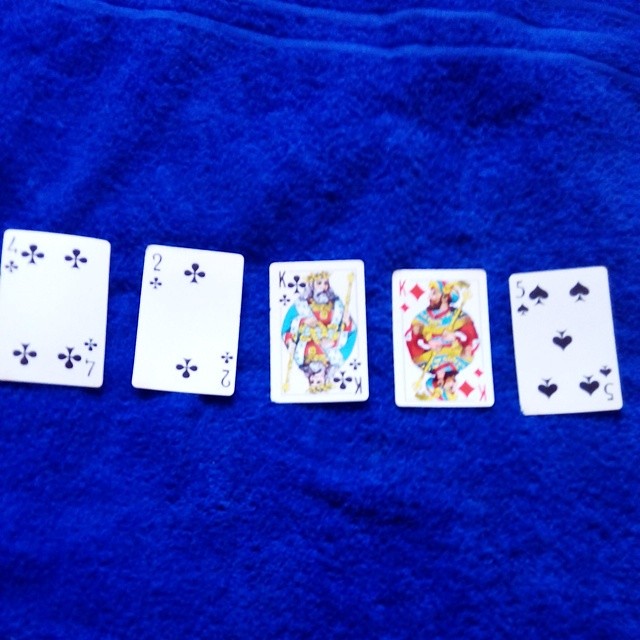A blurry photo captures an array of five playing cards haphazardly arranged on a bright royal blue fleece blanket, characterized by ribbing at the top. Among the cards, starting from the leftmost, is a four of clubs with an unusual, medieval design. Next is a two of clubs, followed by a king of clubs in a striking aqua coat, resembling a crowned, Jesus-like figure. Beside him sits a king of diamonds, depicted as a man in a turban adorned in teal, red, and yellow attire. The sequence ends with a five of spades, completing the horizontal lineup across the soft, textured background.